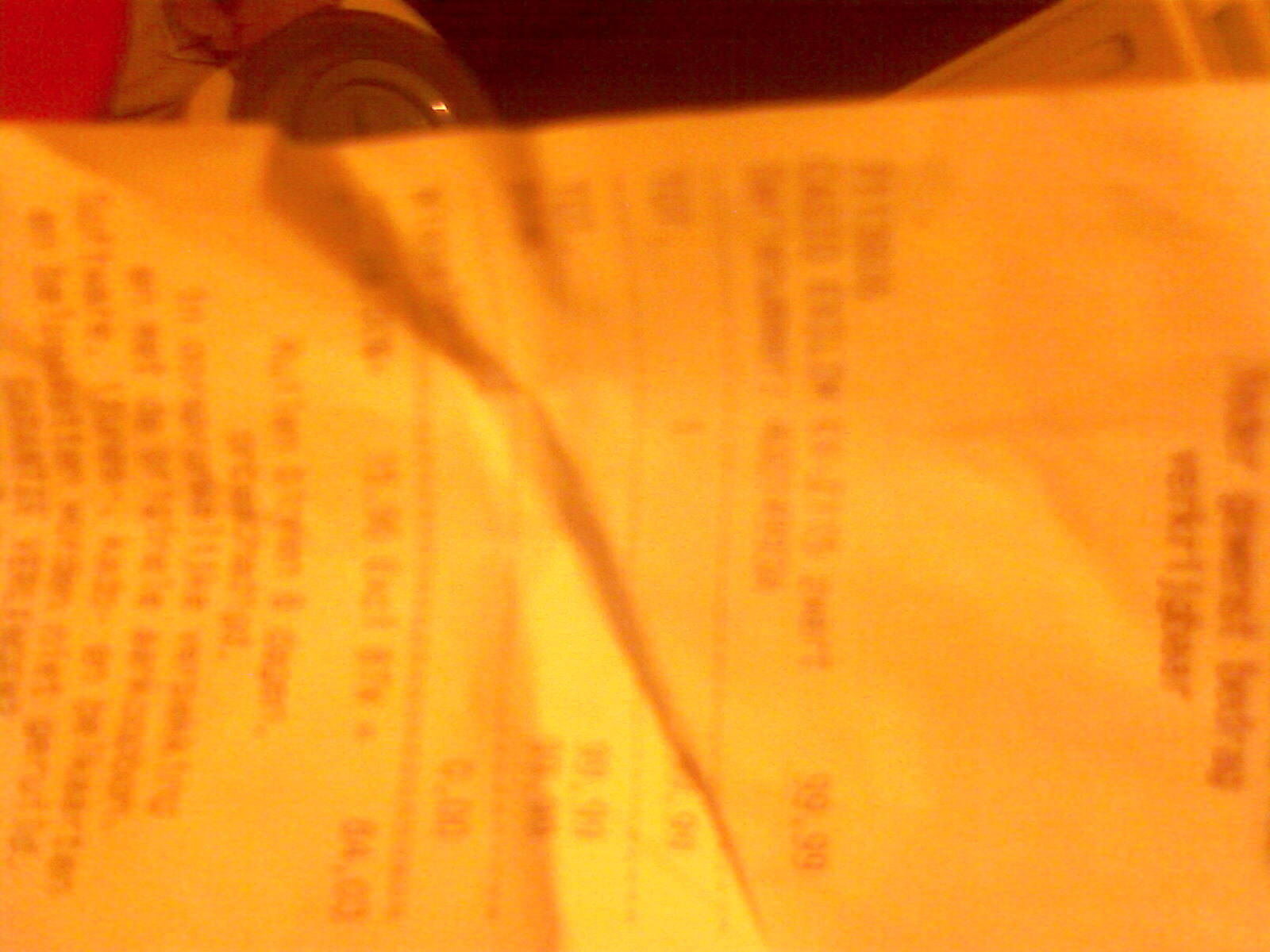The image depicts a crumpled receipt that has been rotated 90 degrees to the right, causing it to be displayed sideways. The photo is notably blurry, with a strong orange tint to the lighting, which makes the text on the receipt hard to decipher. The paper is visibly wrinkled and appears to have been frequently handled and folded. An attempt to make out the details suggests that the total cost is likely 8403, though the specific item and other contents are indecipherable due to the poor image quality. The lower section of the receipt contains some additional text, which is also unreadable.